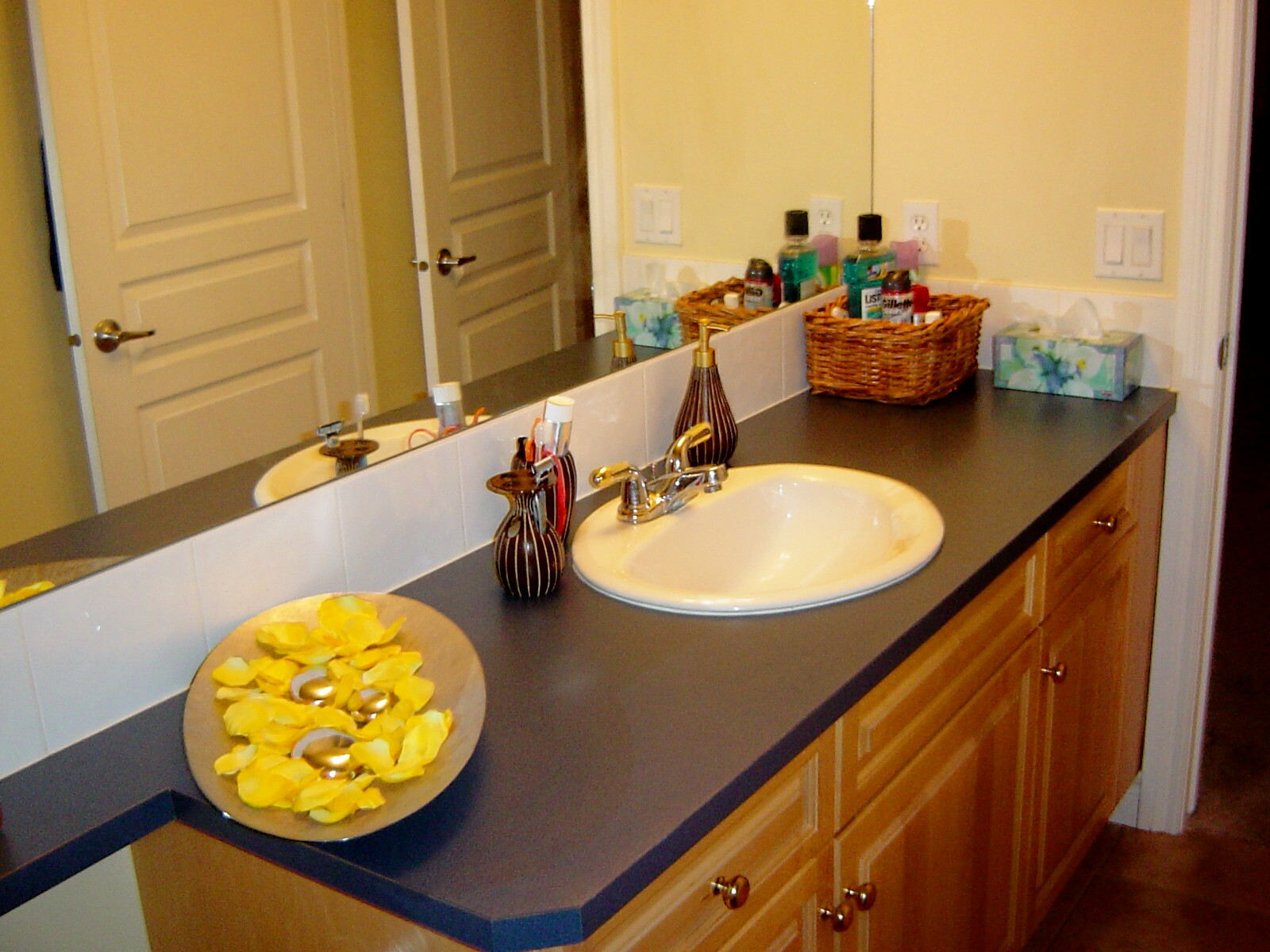A meticulously presented overview shot of a bathroom showcases a brown oak-colored vanity at its focal point. The vanity features brass-colored knobs on both its drawers and cabinet doors, adding a touch of elegance. The dark gray laminate countertop provides a sleek and modern contrast. Positioned on the countertop is a single sink equipped with a dual-tone, silver, and gold faucet. Beside the faucet, a bronze soap dispenser with vertical gold stripes and a gold pump top stands prominently. To the left of this dispenser, a matching bronze vase adorned with similar vertical white stripes complements the ensemble.

The backdrop of the scene is a pristine white tile backsplash, which enhances the overall brightness and cleanliness of the bathroom. Above the vanity, a strikingly large mirror, likely spanning six to seven feet, is mounted on the wall, reflecting the spaciousness of the room. The surrounding walls are painted a creamy white, contributing to a warm and inviting atmosphere. Every element in this image combines to create a detailed and aesthetically pleasing bathroom interior.